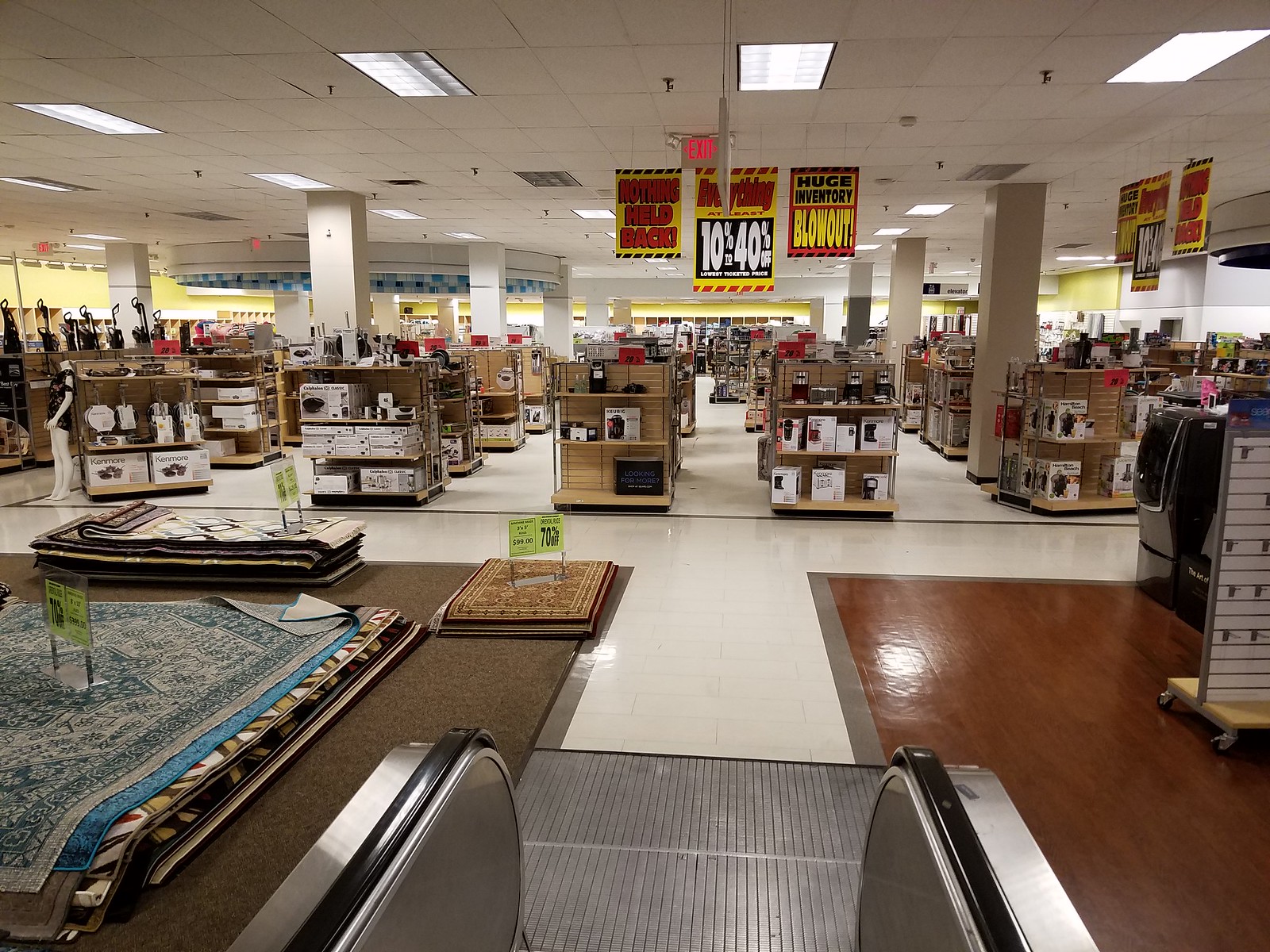The photograph showcases a bustling department store, likely a bargain outlet, due to the plethora of gaudy signs hanging from the ceiling that announce various promotions like "Huge Inventory Blowout" and discounts ranging from 10% to 40% off. The image appears to be taken from the point of view of an escalator situated in the center, although it is unclear whether the escalator is moving upward or downward.

At the end of the escalator, the floor transitions to white linoleum, leading to an intersecting path that branches left and right. Immediately to the left of the escalator is the rug section, featuring stacks of small, medium, and large rugs with vibrant yellow signs indicating a 70% discount on each pile. On the right side of the escalator, the flooring changes to brown, and what looks like a laundry appliance—possibly a washing machine or dryer—can be seen.

Further into the store, there are aisles filled with various goods displayed on racks, likely kitchen items. Some of these items appear to be juicers or coffee machines, although it's somewhat indistinct. To the far left, a headless mannequin stands amidst vacuum cleaner handles. Fluorescent lights on the ceiling illuminate the entire scene, casting a utilitarian glow over the chaotic yet inviting shopping area. Brightly colored signs in yellow and red enhance the lively atmosphere, reinforcing the impression of an energetic, discount-driven shopping environment.